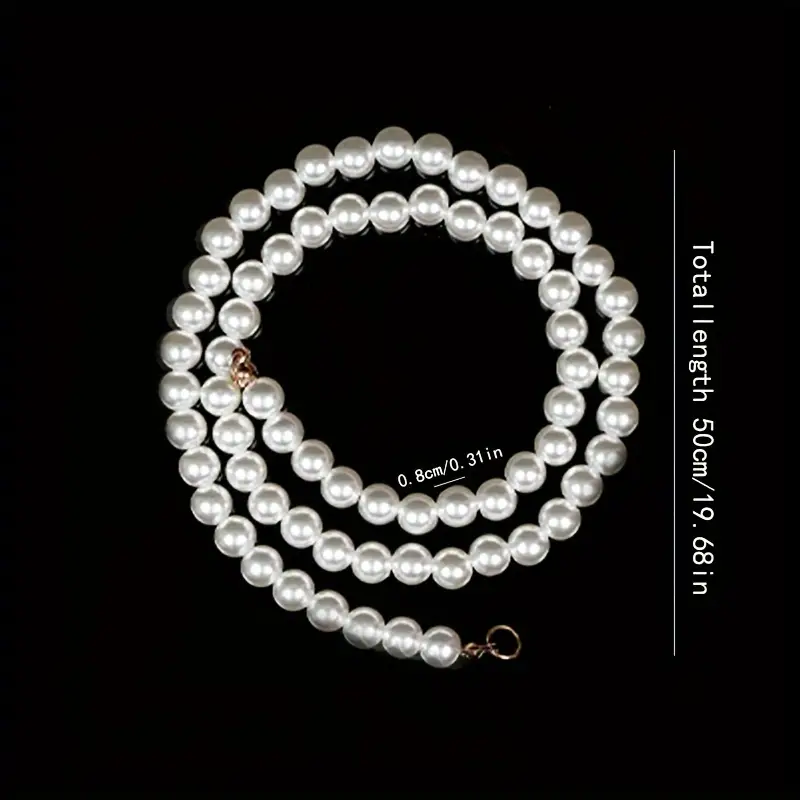This image features a centrally-placed strand of pearls arranged in a coiled, circular pattern against a shiny black background, reflecting the pearls. Each end of the necklace showcases a clasp, one appearing brass or gold, located slightly right of center and below center, and the other positioned at the end of the circular coil. In the middle of the necklace, white text overlays a pearl, reading "0.8 cm / 0.31 inches." To the right of the pearls, a vertical white line with white text alongside it indicates the "total length 50 cm / 19.68 inches." The detailed arrangement and measurements suggest this image is for product display purposes.